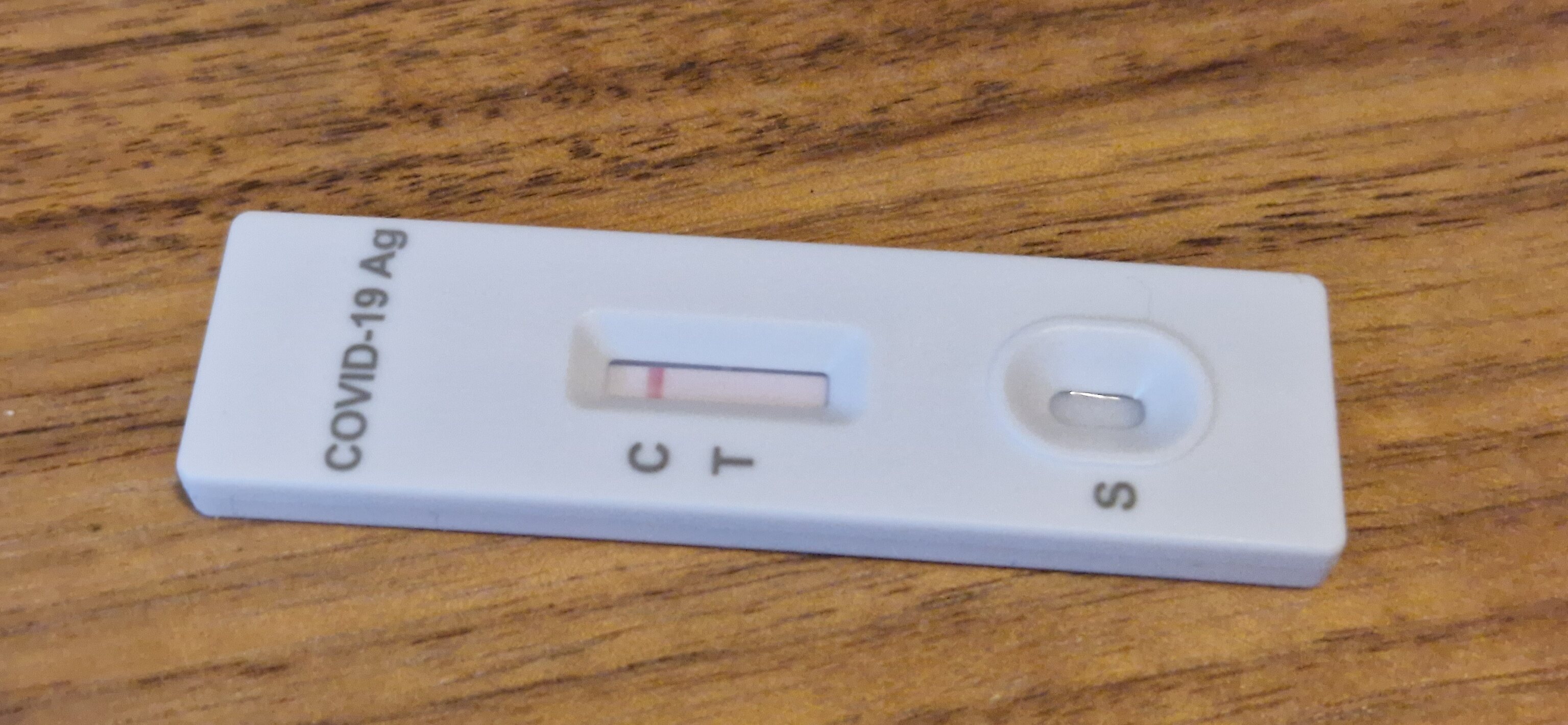A wooden table displaying a striking contrast of light and dark brown grains serves as the backdrop for a COVID-19 antigen test lying horizontally. The table's intricate grain pattern is more pronounced at the top, showcasing heavier, darker wood that gradually transitions into lighter shades towards the bottom. Resting on the surface is a long white plastic test strip, approximately four to five inches in length. The strip features gray lettering at the top spelling out "COVID-19 AG." Below the text is a small window with gray letters "C" and "T" adjacent to it. A red mark is visible next to the "C," indicating the control line. Additionally, an "S" is positioned at the bottom, adjacent to a small oval circle that remains empty. The meticulous arrangement on the table highlights the contrast between the aesthetically pleasing wood grain and the clinical appearance of the test strip.